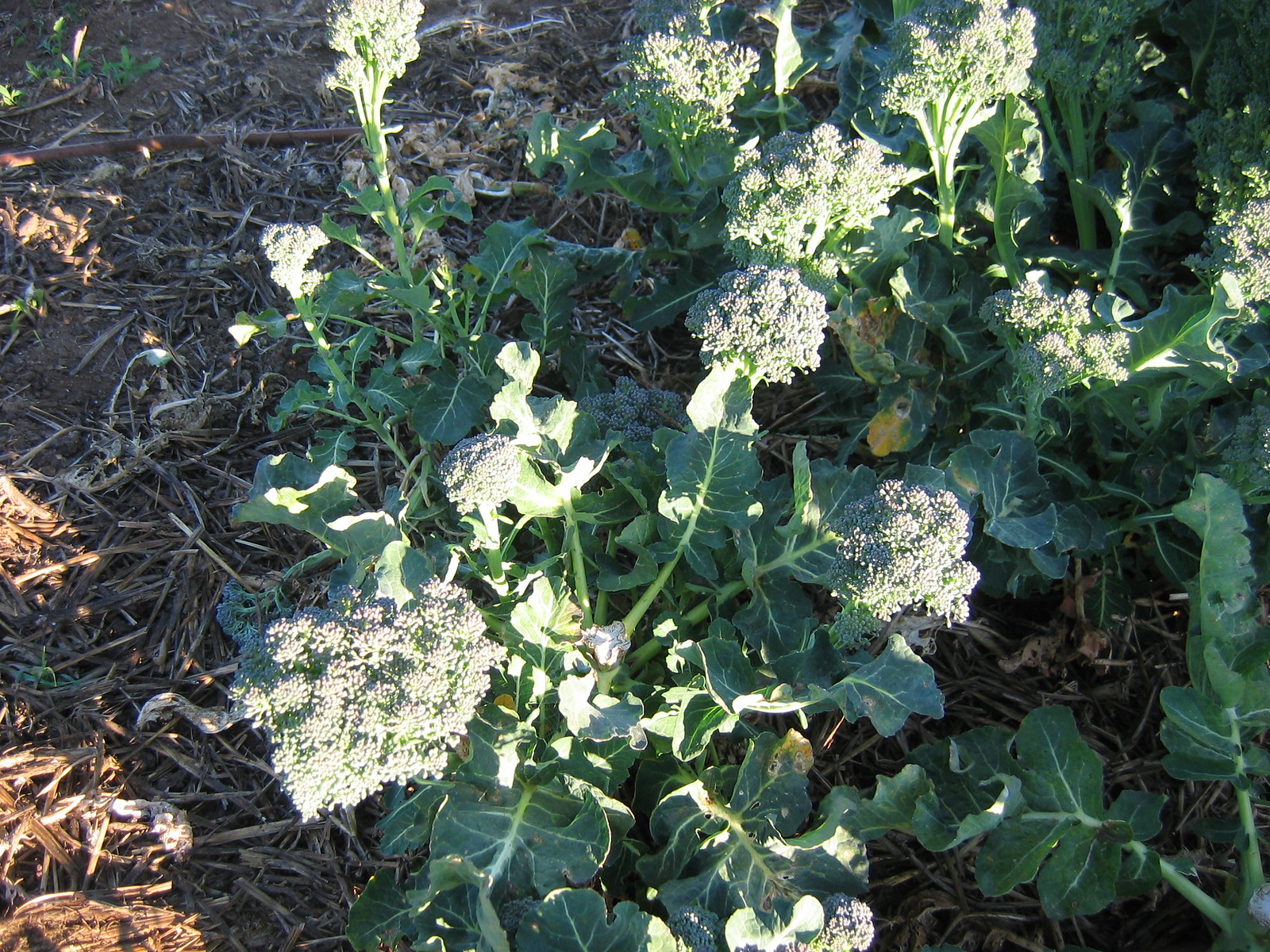This color photograph captures a close-up, straight-down view of a plant bathed in sunlight. At the center, the plant has broad, dark green leaves with lighter green veins, most of which are in shadow. The leaves give rise to white, spherical flower heads that resemble alliums, made up of even smaller, spherical clusters. These delicate flowers, tiny and bright white, are illuminated by sunlight, which makes them appear exceptionally vibrant. Surrounding the plant is a greyish-brown ground covered with what appears to be dead foliage, bark, or mulch, primarily shaded except for areas in the bottom right and left corners where sunlight peeks through, creating a contrasting play of light and shadow on the scene.